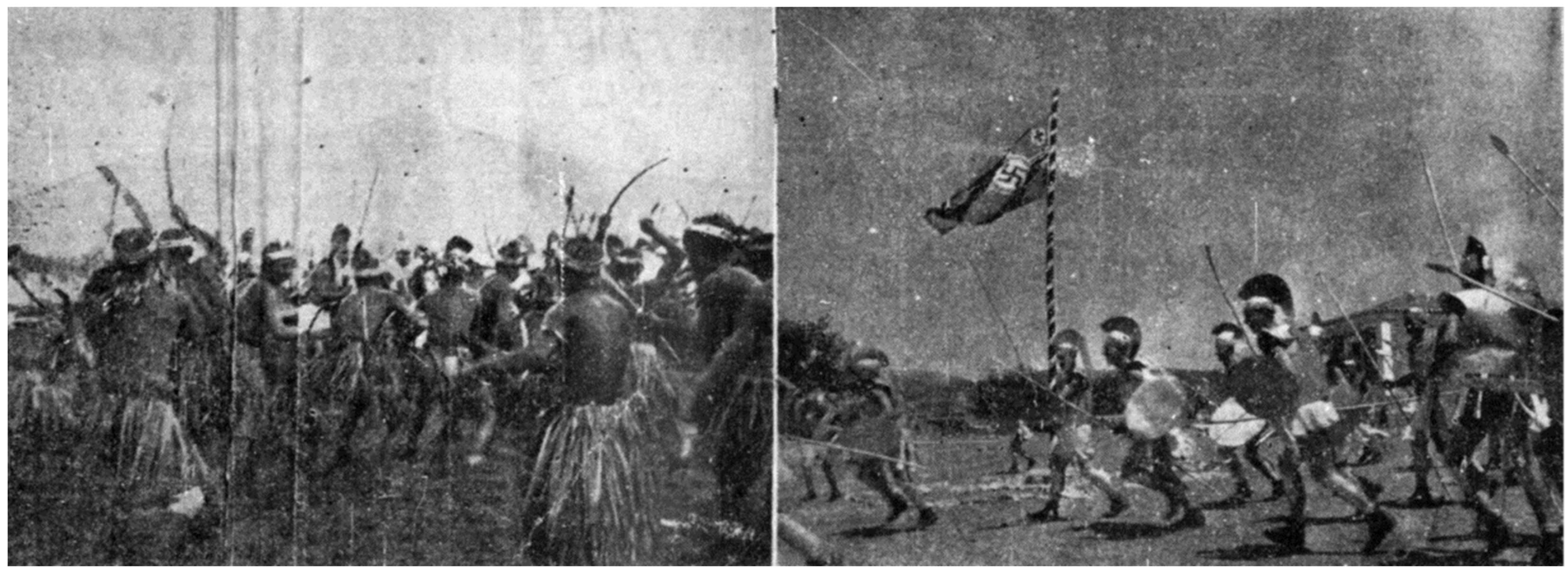In this pair of horizontally oriented black-and-white photographs, the left image, faded and reminiscent of tintype photography, depicts a group of native men from the 1800s or early 1900s, possibly in a Borneo-like setting. These men, adorned in traditional attire including headbands and grass skirts, encircle a central Caucasian man, raising swords and bows above their heads, creating a scene thick with tension and ambiguity, further compounded by mountains faintly visible in the background. The scene is chaotic, suggesting an imminent or ongoing skirmish. In stark contrast, the right photograph, another black-and-white image, appears more recent and captures a dramatic reenactment of a gladiatorial event. Men dressed in Roman or Greek-style warrior costumes, complete with helmets, shields, and spears, engage in combat or perhaps a ritualistic display. The presence of a Nazi flag among these warriors, along with the indication of trees and a hill in the muted background, adds a perplexing historical overlay to the scene. The two images together create a fascinating juxtaposition of historical and recreated battle scenarios, rich with cultural and temporal layers.